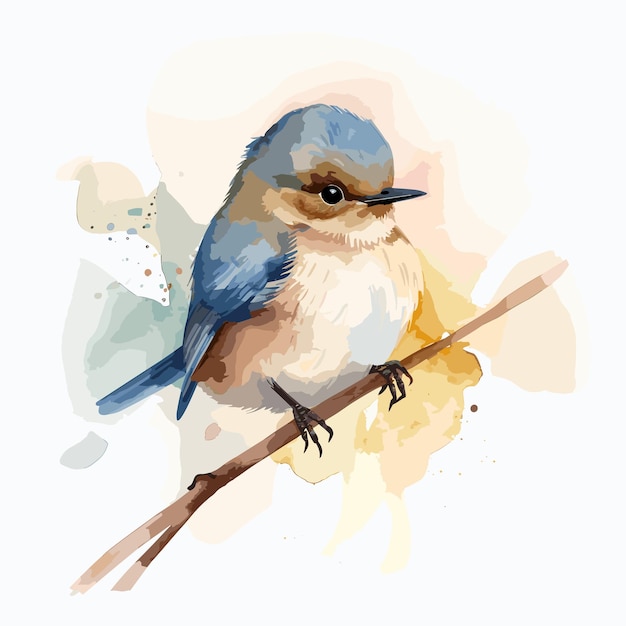This image is a detailed watercolor drawing of a very tiny, baby bluebird perched on a medium-brown twig that angles upwards at 45 degrees from the left-hand corner of the frame. The bird is facing to the right, its beak, a black or dark gray color, is closed as it looks intently at something off-frame. The bluebird flaunts a mix of blue feathers on the top of its head and wings, with its breast and belly showcasing shades of white, tan, and light brown. There are additional darker brown hues around its neck and under the wings. Its black feet are clearly visible, grasping the branch firmly, showcasing each toe distinctly. The background features an indistinct blend of watercolor shades—white, pale tan, light green, and hints of pink—creating a subtle, puddle-like effect that draws focus onto the bird.